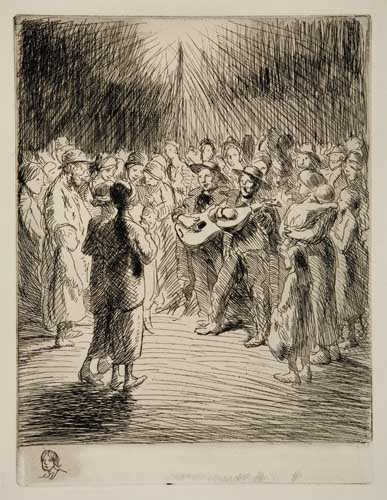This detailed pencil sketch depicts a lively scene of a singing group amidst a gathering. Central to the image are two front singers, their mouths open in mid-song, with their backs to the viewer. Among the audience, which includes men, women, and children, two men stand out, each strumming an acoustic guitar and wearing black jackets and pants. The audience's attentive gaze is fixed on the performers, creating an atmosphere of celebration. On the right side of the crowd, a woman in a dress holds a sleeping child, while nearby, a small girl with long brown hair, likely around six or seven years old, stands alone. The sketch's background is interspersed with lines that suggest either a ceiling or an open sky, complementing the sunlit ambiance. Additionally, hints of trees or bushes are drawn, adding depth to the scene. The image is bordered by a white frame, and there is a name at the bottom, though it is blurred and unreadable. The overall tone of the sketch is black and white with some light green coloring due to the paper quality, adding a timeless, serene quality to this celebratory gathering.